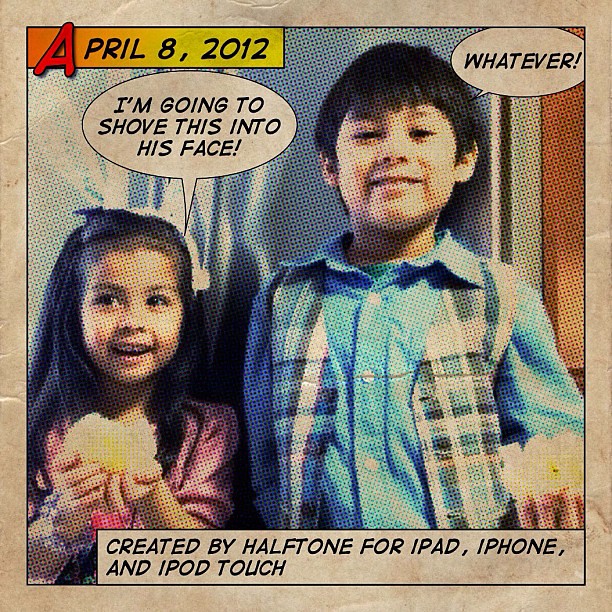The image is a playful, comic book-style photograph featuring a young girl and a slightly older boy. The girl, dressed in a pink outfit, is smiling and holding up an indistinguishable object, possibly a piece of cloth, while the boy, wearing a blue shirt with a plaid vest, stands next to her, also smiling. At the top left corner, there's an orange-yellow rectangle with the date "April 8, 2012" in red and black text. Speech bubbles add a humorous touch, with the girl’s bubble stating, "I'm going to shove this into his face," and the boy’s bubble simply saying, "whatever." In the bottom right corner, a caption reads, "Created by Halftone for iPad, iPhone, and iPod touch," in black text.